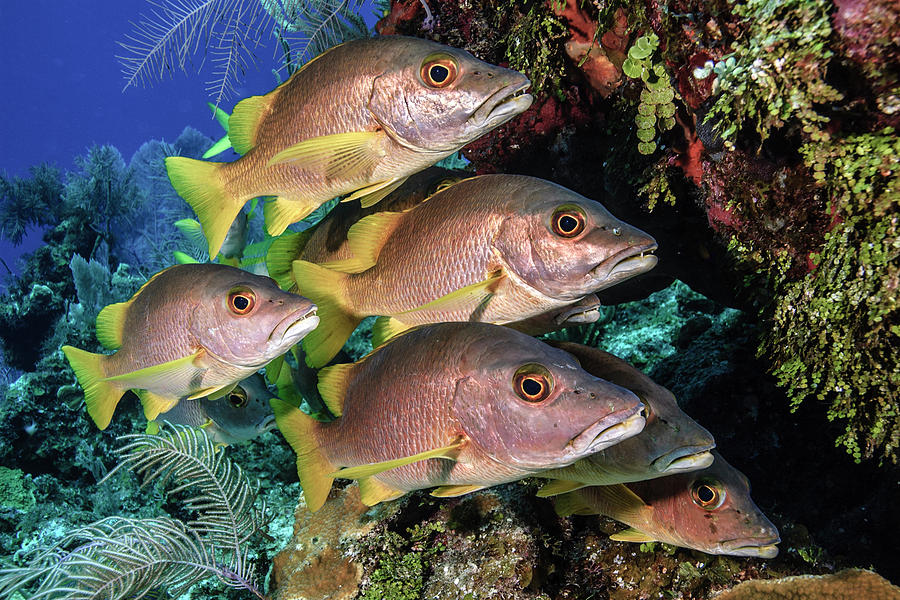This underwater photograph captures a small school of six light golden, silver-metallic fish with strikingly bright yellow fins and tails. The fish, shown from a side view, appear to be swimming upwards and are characterized by their large eyes, which have dark black pupils surrounded by a copper and yellow ring. Some of the fish have their mouths slightly open, revealing fairly sharp teeth. They are gracefully moving in and out among the lush underwater vegetation and rocky outcrops, which might be coral. The reddish rock formations in the background are adorned with green underwater plants and moss. The surrounding water is a vibrant blue, highlighting the diverse sea life and additional coral growing from the ocean floor. The fish seem almost to engage with the viewer, each looking directly at the camera as they glide by, under the illuminated light that enhances the scene's natural beauty.